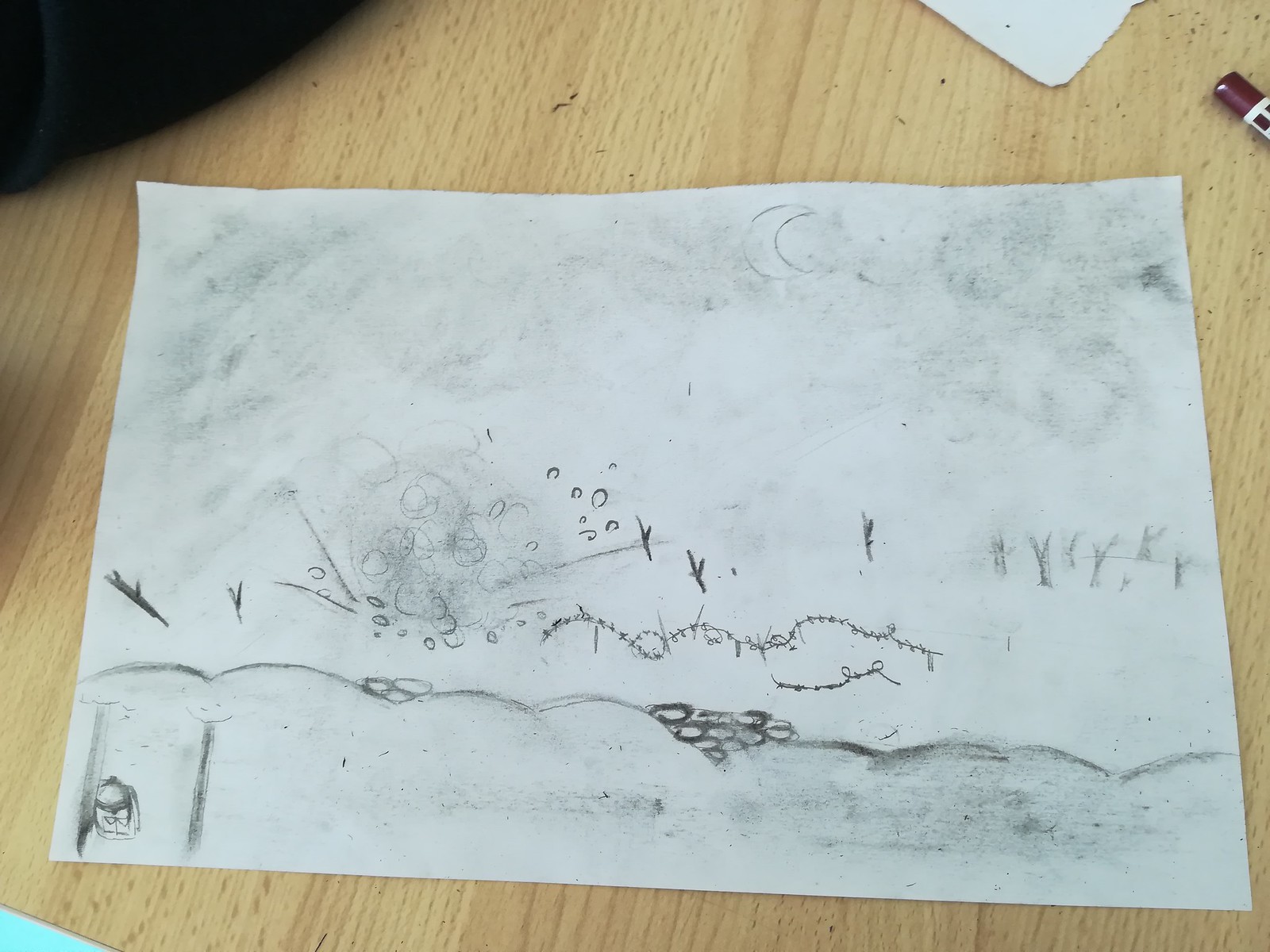This close-up image features a piece of white paper lying horizontally on a light, tan, wood grain laminate surface. The paper is filled with numerous small jottings, made with both pencil and black ink, some of which are smudged. Approximately a quarter of the way from the bottom, there is a series of eight small, arch-like humps that stretch from the left side to the right. Within one of these humps are three small ovals resembling rocks. In the deepest hump, there are about eleven similar ovals clustered together. Beneath these humps, there's additional pencil smudging.

On the left-hand side of the paper, there are two vertical lines adjacent to a drawing of a head with a bandana, triangle eyes, and a straight mouth. Above these humps in the center, several little X's form three more humps. These X's, along with other tiny, hard-to-read scribbles, add to the playful, scribbled nature of the page.

To the left of the paper, separate clusters of small rocks, a stick, and the letter 'Y' can be seen. There are also three more 'Y' shapes, which appear to represent trees. On the right-hand side, there are six faint 'Y' shapes, reinforcing the tree-like imagery.

At the top, just to the right of the center, a crescent moon resembling the letter 'C' is visible. The upper portion of the page shows a significant amount of smudging, likely from someone with graphite on their fingers, contributing to the overall messy and organic feel of the drawing.